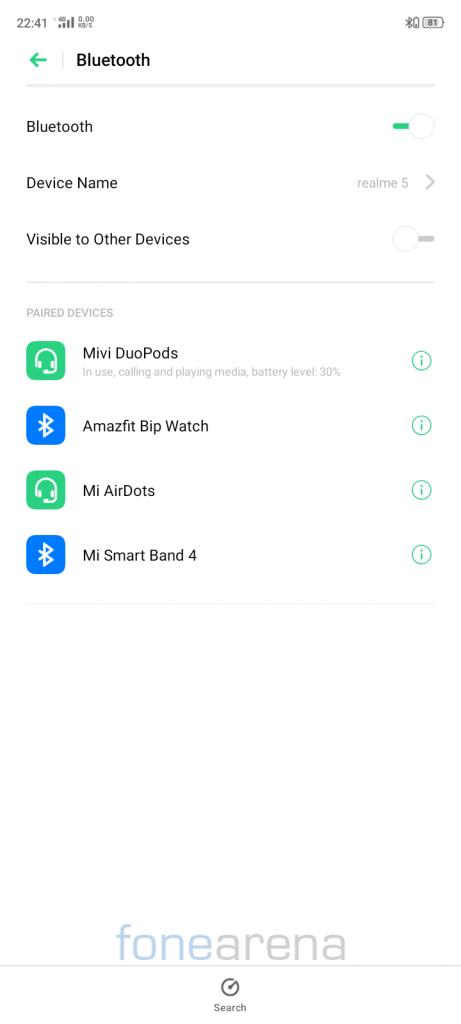The image displays a digital interface with various icons and text. At the top, the time "22:41" is visible alongside four black bars of varying heights, indicating signal strength. Below these, there are two lines of numbers too small to decipher.

To the right, a Bluetooth icon and a vertical battery icon are present. Adjacent to these is a gray rectangle that likely reads "81". 

The next section features a left-pointing green arrow and a vertical gray bar with the word "Bluetooth" in bold letters. Following this is a gray horizontal bar extending across the screen. Beneath this bar, "Bluetooth" is written again, accompanied by a green slider with a white button, indicating Bluetooth is enabled.

The subsequent line displays "Device Name: realme 5" with a right-pointing arrow. Below, the text "Visible to other devices" appears beside a gray slider with a white button, showing this option is disabled.

A horizontal gray line separates sections, leading to "Paired Devices". Here, a green square with headphones and a speaker icon appears, labeled "MIVI DuoPods in use, calling and playing media, battery level 30%". 

Lastly, a green outline circle features an upside-down exclamation mark, followed by a blue square with the Bluetooth symbol, completing the detailed view of the interface.